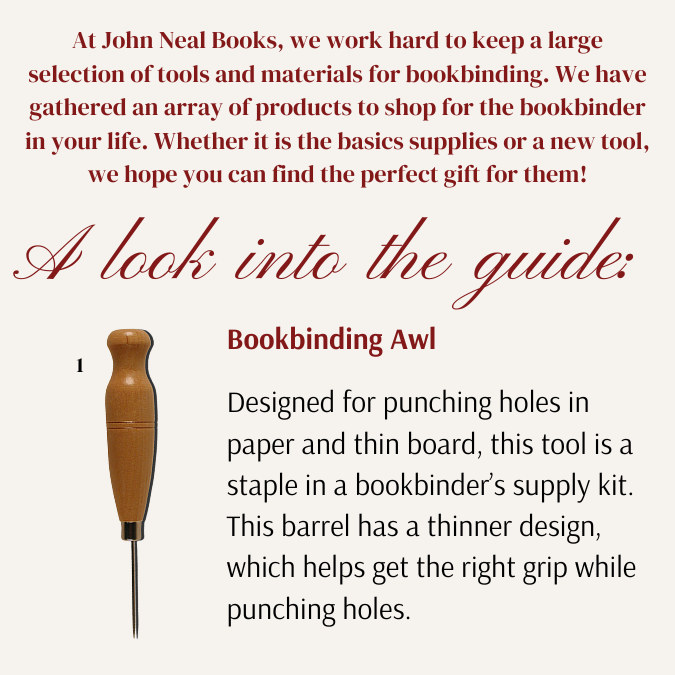The image is an advertisement poster set against a light pink background, featuring a red and black script title, "A Look into the Guide," in the center. Below the title, in cursive, it reads "Bookbinding Awl," with an accompanying photograph to the left of a wooden-handled awl, resembling a screwdriver with a metal tip designed for punching holes in paper and thin board. This essential tool for bookbinding has a thinner barrel for improved grip. The top of the poster contains a red text paragraph explaining, "At John Neal Books, we work hard to keep a large selection of tools and materials for bookbinding. We have gathered an array of products for the bookbinder in your life, whether it’s basic supplies or new tools. We hope you can find the perfect gift for them." The lower right corner includes a detailed description of the awl: "Designed for punching holes in paper and thin board. This tool is a staple in a bookbinder’s supply kit. The barrel has a thinner design, which helps get the right grip while punching holes."